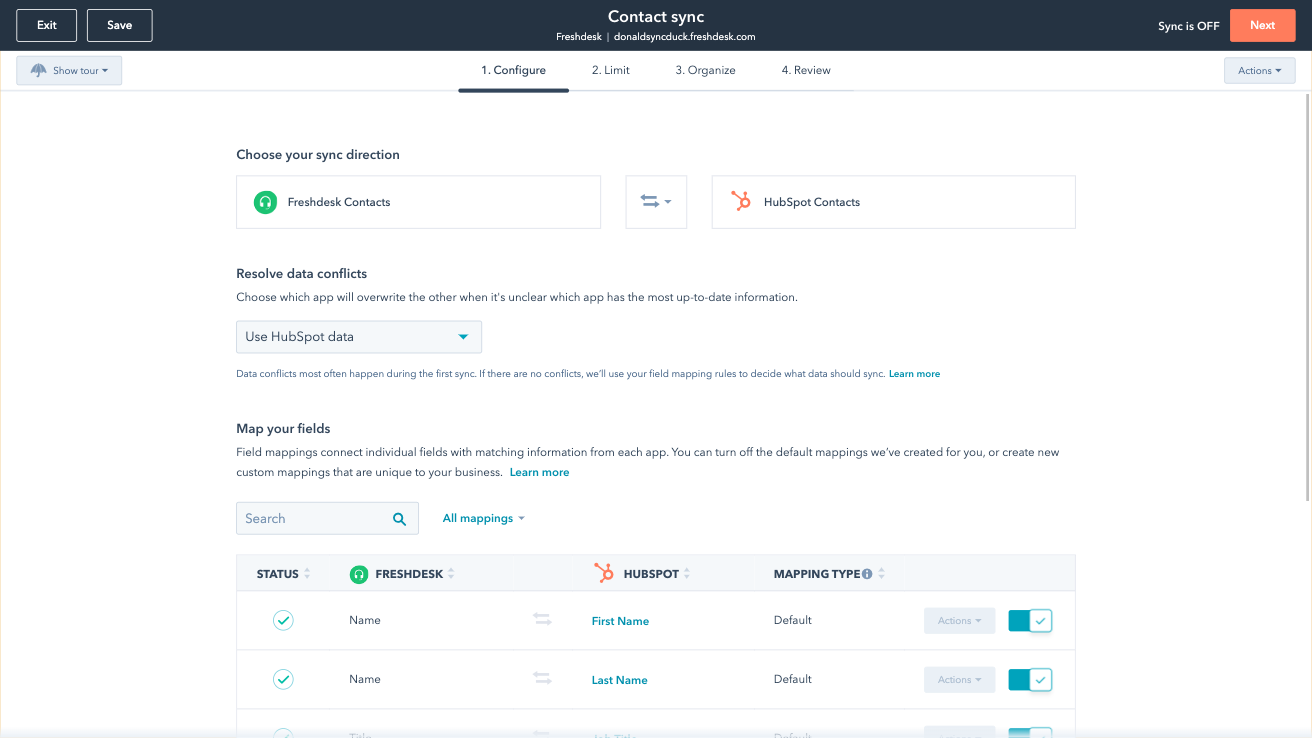The image depicts a "Contact Sync" interface page. At the top left corner, there are "Exit" and "Save" buttons, presented in white font within a white box on a black background. This header spans the width of the image, and centrally placed within it is the title "Contact Sync" in larger font. Beneath that, in a smaller font, the URL "freshdesk/donalds-sync-doc.freshdesk.desk.com" is displayed.

On the right side of this header bar, it states "Sync is off" followed by a "Next" button. Below this, there are four tabs labeled "Configure," "Limit," "Organize," and "Review," with the "Configure" tab being selected.

Under the "Configure" tab, several configuration options are presented. These include:
1. "Choose your sync direction"
2. "Resolve data conflicts"
3. "Map your fields" 

Each section provides various controls and settings. At the bottom, there's a set of toggle buttons corresponding to different platforms such as "Freshdesk," "HubSpot," and a column titled "Mapping Type."